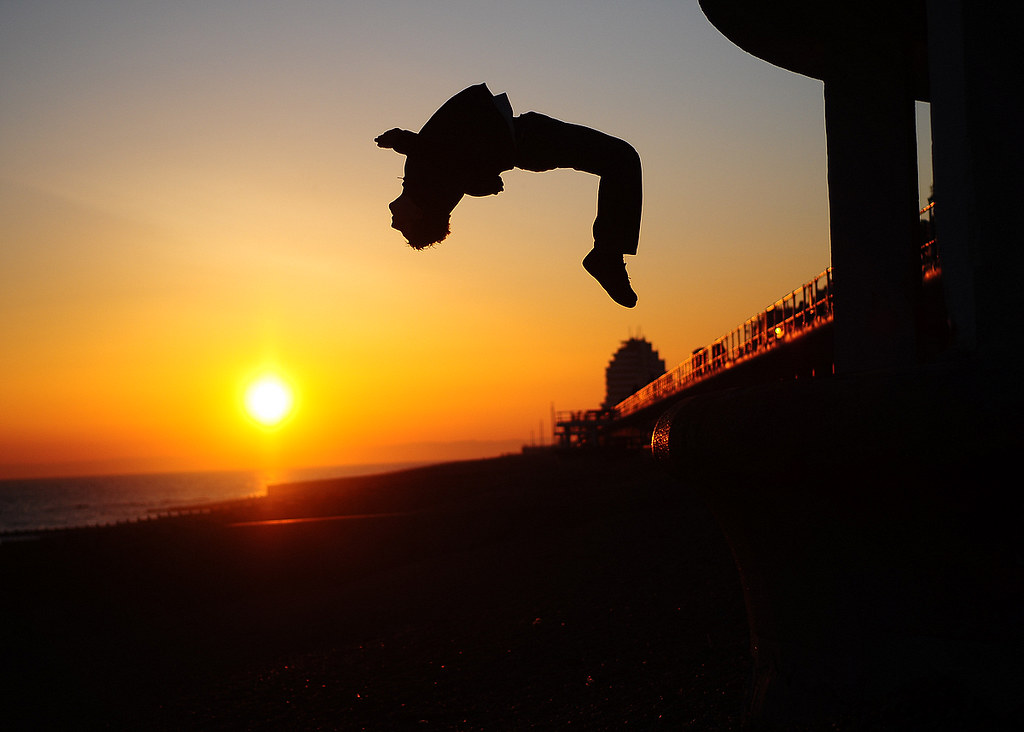The photograph captures a striking outdoor scene set at a beach during a vibrant sunset. The top of the image is dominated by the sun, which is almost fully set, casting a brilliant yellow and orange glow across the sky. The sun's reflection creates a shimmering pathway on the water below.

In the foreground, a man, silhouetted against the radiant backdrop, is captured mid-air in the midst of performing a backflip. His body arcs gracefully, with his feet trailing behind and his head bent downward in a perfect half-flip. The silhouetted figure, dressed in jeans, a coat, and shoes, stands out starkly against the bright sky, his short hair noticeable even in the shadow.

The scene is framed by a few key elements: a guardrail near the water, a line of pilings suggesting a pier, and a silhouetted column to the right, possibly part of a larger structure. The dark silhouettes of these elements contrast sharply with the bright, colorful sky, adding depth and context to the dynamic moment of the man’s jump.